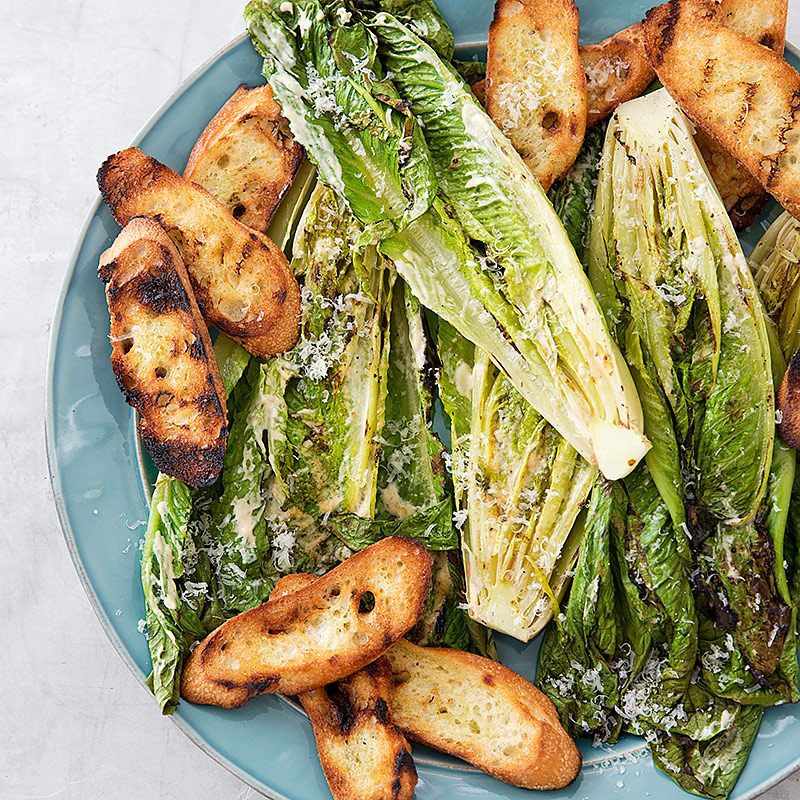This square color photograph, taken indoors from a top-down perspective, showcases a large, round blue plate overflowing with a savory blend of grilled and baked ingredients. Occupying most of the plate, the centerpiece is halved stalks of romaine lettuce, their once verdant leaves now browned and curled from grilling. The charring imparts a rustic look, with hints of golden-brown edges and some blackened tips. A generous sprinkling of shredded white Parmesan cheese coats the lettuce, adding a rich contrast.

Surrounding the lettuce, there are long, thin strips of garlic bread, equally grilled, displaying a spectrum of colors from golden brown to charred black. The inside of the breadsticks reveals a creamy white interior. The plate's vivid blue, occasionally peeking through the food, enhances the visual appeal against the light gray stone countertop beneath, which features subtle darker striations. The composition suggests a satisfying rustic meal with a unique twist, highlighting both the hearty grilled lettuce and the crisp, savory garlic bread.